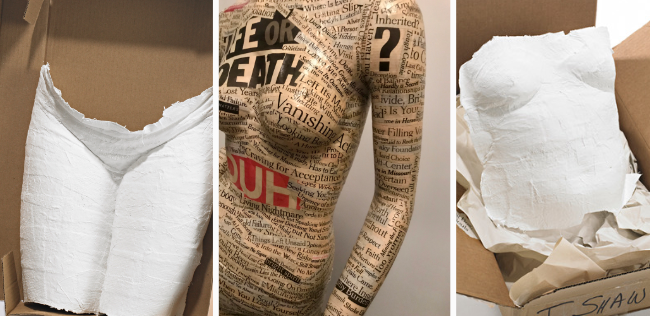The color photograph collage displays three detailed, end-to-end images arranged horizontally that portray the process and results of papier-mâché art focused on the human female form. On the far left, the first image features a white plaster cast of the lower female torso, extending from just above the knees to just below the waist, laid out on a piece of cardboard. The central image showcases a full female torso, from the shoulders to the hips, meticulously covered in yellowed newsprint, adorned with black text featuring words like "life or death," "vanish," and a question mark, against a subtly aged background. The rightmost image depicts another paper mâché or plastered torso, focused on the female chest down to the belly button. This piece is also white, packaged with crepe and laid atop brown packaging paper, creating a visually cohesive and intriguing exploration of form and material, likely indicative of a fashion student's creative work with varied textures and media on body shapes.